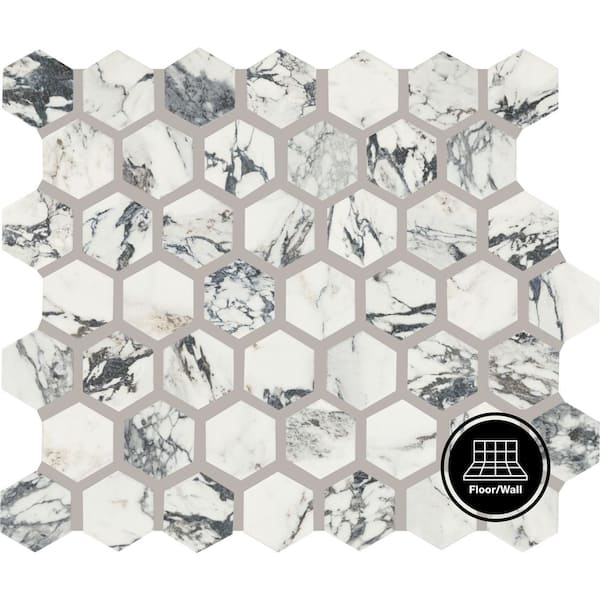The image showcases a detailed marble-patterned flooring or wall section, overlaid with an interlinked honeycomb grid composed of pentagons. The grid, drawn in a light gray shade, overlays a black and white marble texture, complete with swirling veins of gray and black. In the upper left corner, there appears to be an image of a person in bulky clothing within one of the pentagons. At the bottom right, a distinct black circle outlined by a white ring and another black ring encloses a logo. This logo features a stylized representation of flooring and wall, depicted by squares shrinking with perspective to distinguish floor from wall. Beneath the image, the text "floor/wall" is written in white against the black background. The overall composition suggests a sample of a home installation material, such as flooring or wallpaper.